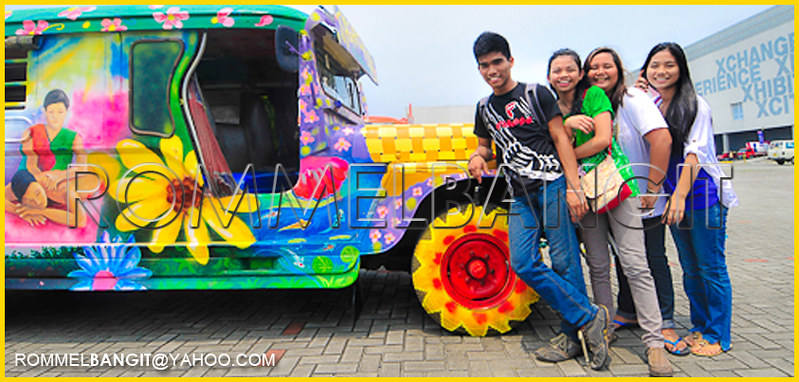This horizontally aligned rectangular image, framed with a yellow border, captures a group of four smiling teenagers—three young women and one young man—posing by the vividly painted front end of an old-styled car, possibly a Jeep. The vehicle is adorned with a colorful mural featuring large flowers, including daisies, checker patterns, and a depiction of a woman massaging someone. The palette includes bright greens, pinks, purples, blues, and a front tire whimsically painted yellow with an orange sun in the center. 

The first teenager, a young man with dark hair, wears a patterned black-and-white t-shirt paired with blue jeans. Beside him stands a young woman in gray pants, a bright green shirt, and carrying a purse. Another young woman sports a white t-shirt, blue jeans, and flip-flops, while the last individual, with long pretty dark hair, mirrors her outfit but with rolled-up sleeves. They are all standing outdoors on a partly cloudy day, with a building featuring blue symbols visible in the background, suggesting the scene is likely set outside of America.